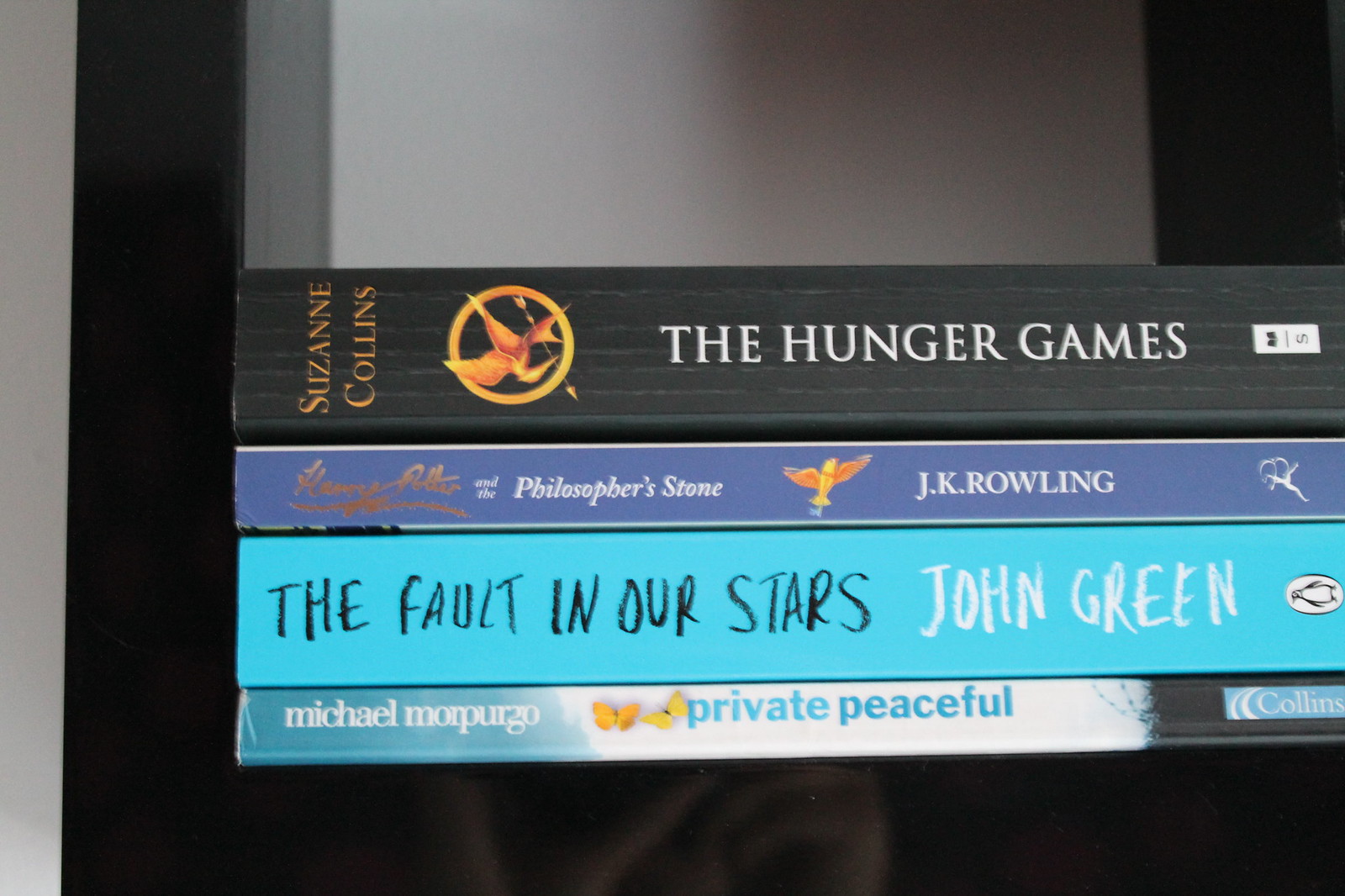The image features a stack of four books lying flat on a black bookshelf against a white wall. From top to bottom, the books are: "The Hunger Games" by Suzanne Collins, with a black cover and orange and white text; "Harry Potter and the Philosopher's Stone" by J.K. Rowling, with a blue cover and white lettering; "The Fault in Our Stars" by John Green, with a turquoise spine and black and white text; and "Private Peaceful" by Michael Morpurgo, with a half turquoise, half white spine and turquoise letters. Notable details include the presence of specific animals on the book covers: a mockingjay on "The Hunger Games," an eagle on "Harry Potter," and a penguin on "The Fault in Our Stars."